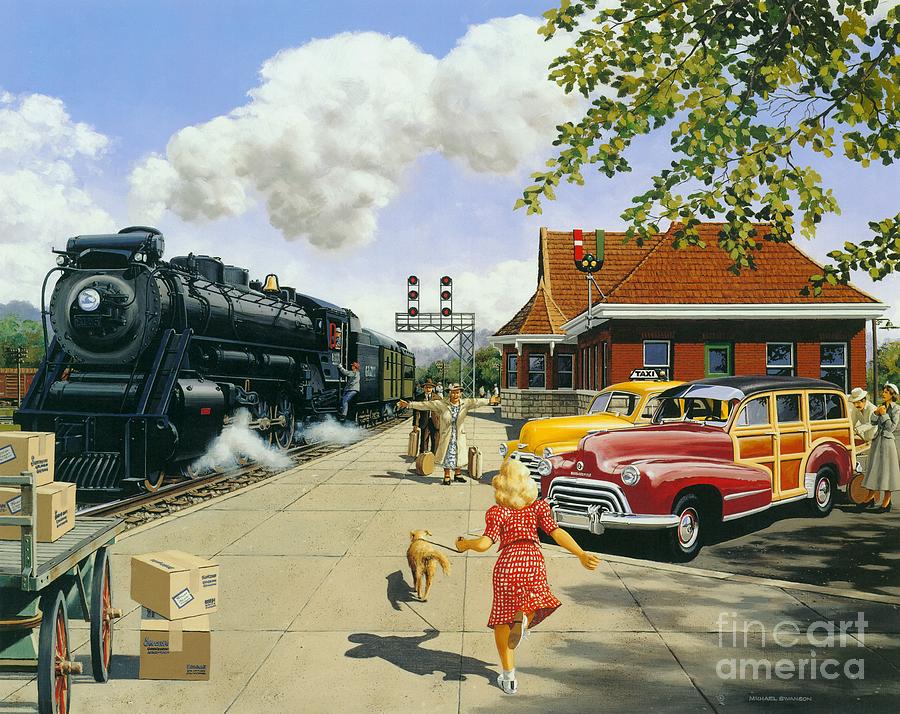This painting portrays a touching scene at an old-fashioned train station, with meticulous details evoking a nostalgic atmosphere. It features a young girl, perhaps around 12 to 14 years old, prominently positioned at the bottom center of the image. She has blonde hair and is dressed in a red and white checkered dress. Captured in mid-run, she is seen from behind, and her left hand clutches the leash of a small brown dog that bounds ahead of her. She casts a shadow to her left and forward as she rushes towards two figures in the center.

The two adults she is running towards appear to be her grandparents. The woman, joyous with outstretched arms, wears a light tan overcoat over a blue and white patterned dress that falls to her ankles, and she is accessorized with black shoes and a hat. Beside and slightly behind her is a man in a brown suit, also wearing a hat, holding a suitcase in his right hand. A couple of suitcases sit beside the woman, suggesting they might have just disembarked from the train.

On the left side of the painting, a large black steam engine with an old-fashioned cowcatcher is seen at the station, with its coal tender trailing behind. The brown station building with green window sashes and a tiled roof stands to the right. The station platform features an L-shaped railroad signal with red and green flag indicators raised. In front of the station, two vintage vehicles are parked: a large yellow taxi and a red station wagon, possibly from the 1940s or 50s. To the bottom left, a wooden cart topped with stacked cardboard boxes can be seen.

The sky above is a mix of blue and clouds, with some tree leaves peeking in from the upper right corner. Text reading "Fine Art America" is subtly placed in semi-transparent white in the bottom right corner, completing this richly detailed and heartwarming scene.